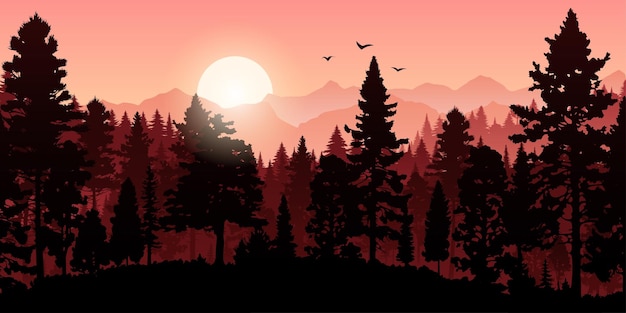The computer-generated image is a horizontally aligned rectangular illustration depicting a serene sunset scene. The top portion of the image showcases a beautiful, peachy-pink sky with a partially hidden, circular yellow sun setting behind a range of mountains, which also appear tinged with pink. Silhouetted against the colorful sky are three birds flying in a distinct 'V' formation. Occupying most of the middle and bottom sections of the illustration, there is a series of pine trees of varying heights. The tallest trees are positioned on the far left and right sides of the image, while the trees in the center are shorter. Additionally, there are multiple layers of tree silhouettes, each layer progressively lighter in color, transitioning from black to dark burgundy, to a lighter red, and finally to a peachy hue. The ground at the bottom of the image is depicted as a solid black, jagged-edged area, emphasizing the silhouetted effect of the trees as they stand against the brightly colored, illuminated backdrop. This vivid and detailed digital landscape, though not realistic, maintains a clear and captivating clarity that beautifully captures the gentle ambiance of a sunset.